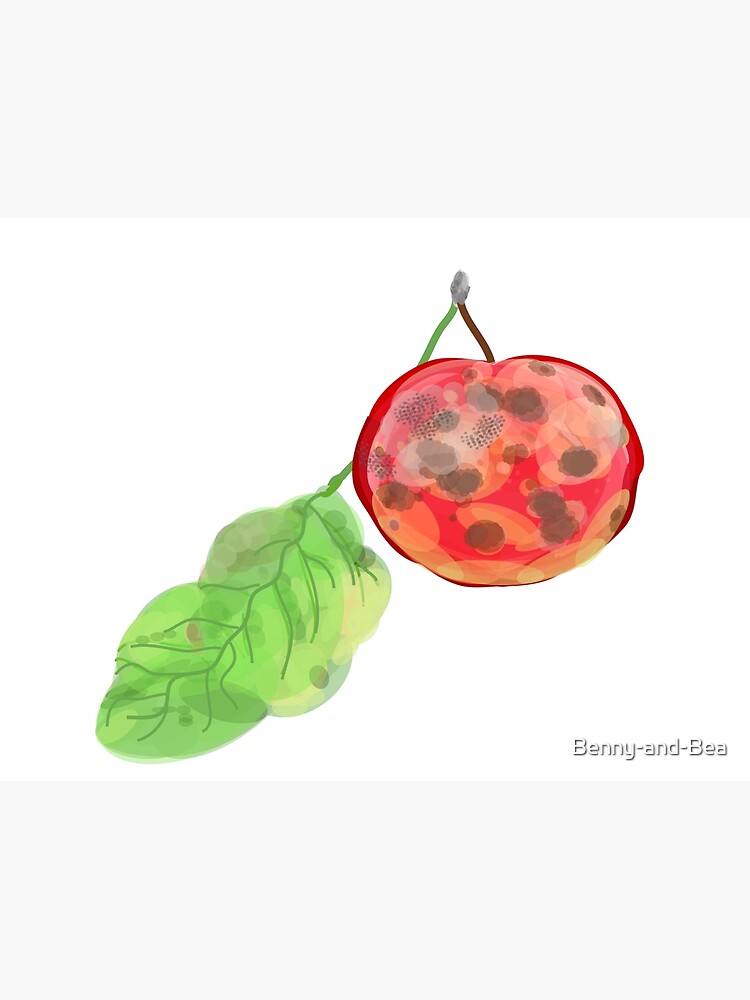This image is a detailed painting that possibly utilizes watercolor techniques. It features a piece of red fruit that most resembles a cherry, although there is some ambiguity, making it could also be mistaken for a strawberry or even an apple. The fruit has noticeable brown spots, suggesting it's somewhat aged or bruised. Extending from the top of the fruit is a stem, which is connected to another stem that supports a green leaf. The leaf is detailed, with prominent green veins and its own patches of brownish and gray discoloration. The background of the image is a plain white, framed by gray rectangles at the top and bottom. The bottom left corner of the image includes the text "Benny and B" in capitalized letters, which appears to be the name of either a business logo or an artist signature. The exact spelling of "B" is unclear but could be "B-E-E" or "B-E-A".